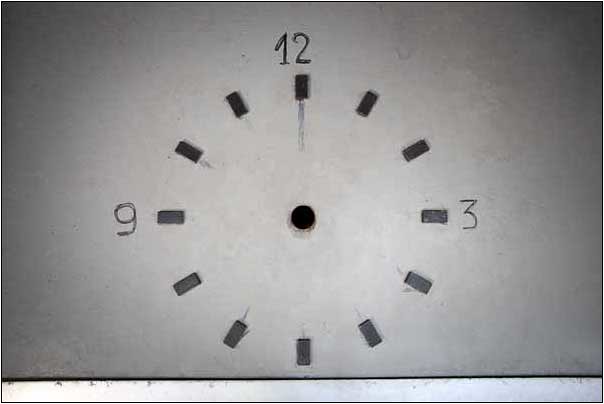This image showcases a close-up of a clock face that appears either drawn or as part of broken clockwork, set against a dirty, bluish white background. The clock face is marked with the numbers 12 at the top, 3 on the right, and 9 on the left, while the remaining hour marks are indicated by small black rectangular bars positioned at 5-minute intervals. The center features a black circular area where the clock hands would typically be attached, but no hands are present. Below the clock face, a thin white bar cuts across the image, with a stark black line running horizontally above it. Additionally, shadowy smear marks can be seen at the 12, 10, and 7 o'clock positions, contributing to the graffiti-like, weathered appearance of the piece. The bottom edge presents a further boundary where the wall or surface turns into a different texture or meets the ground, perhaps adding to the unfinished aesthetic of the artwork.